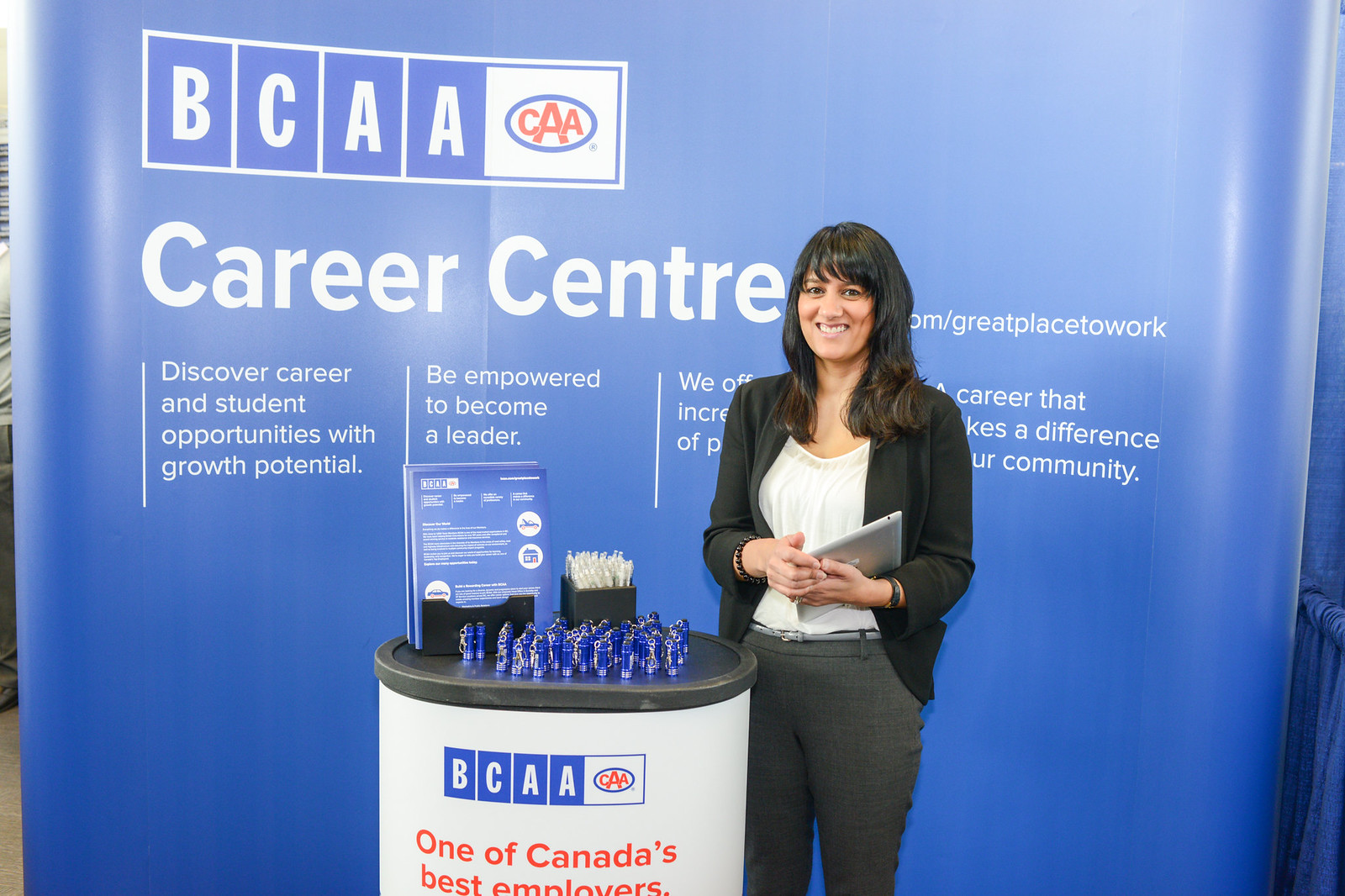A middle-aged Caucasian woman with long, dark brown hair stands in the center of the image, occupying about 70% of the frame from her knees up. She is dressed in business casual attire, wearing a black blazer over a white blouse and gray pants, accessorized with a thin gray-blue belt. She is holding an iPad in her left hand and has her hands gently folded in front of her, smiling warmly. In front of her, there is a white table with a black top displaying the BCAA and CAA logos, along with a sign that reads "One of Canada's Best Employers." The table is adorned with various handouts, including blue pamphlets, small blue flashlight keychains, and other promotional items. Behind her, a large blue banner prominently features the BCAA logo and the CAA insignia. The banner's text includes motivational phrases such as "Career Center," "Discover Community and Student Opportunities with Growth Potential," and "Be Empowered to Become a Leader." The setting appears to be part of a career center presentation aimed at attracting potential employees and students.